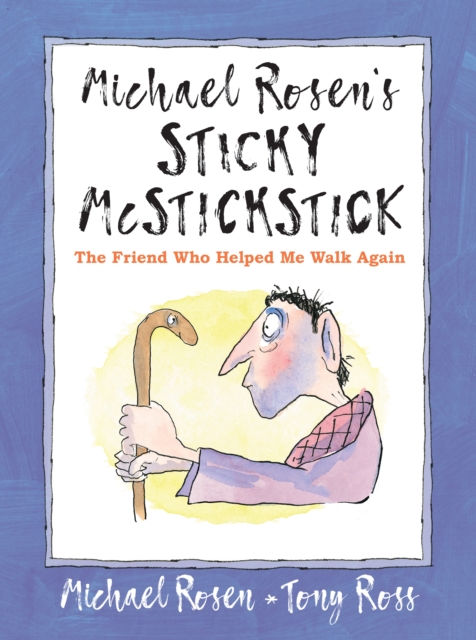The image presents a book cover designed in a digital medium, featuring a striking periwinkle blue border with a subtle gray trim. Dominating the center is a large white rectangle which houses the title and authors' names. The text at the top of the white section is printed in black, stating "Michael Rosen's Sticky McStickstick." Below this, in a vibrant orange font, it reads, "The Friend Who Helped Me Walk Again." At the very bottom of the blue border, white cursive text credits Michael Rosen and Tony Ross.

An illustration below the title on the white background depicts an elderly man with a pale complexion, exaggerated features including a large ear and long nose, and dressed in a red robe. He appears to be in a state of contemplation or exhaustion, intensely staring at his walking cane. The cane is brown and uniquely designed to resemble a snake, complete with an eye and a small mouth, giving it a lifelike appearance as it gazes back at the man.